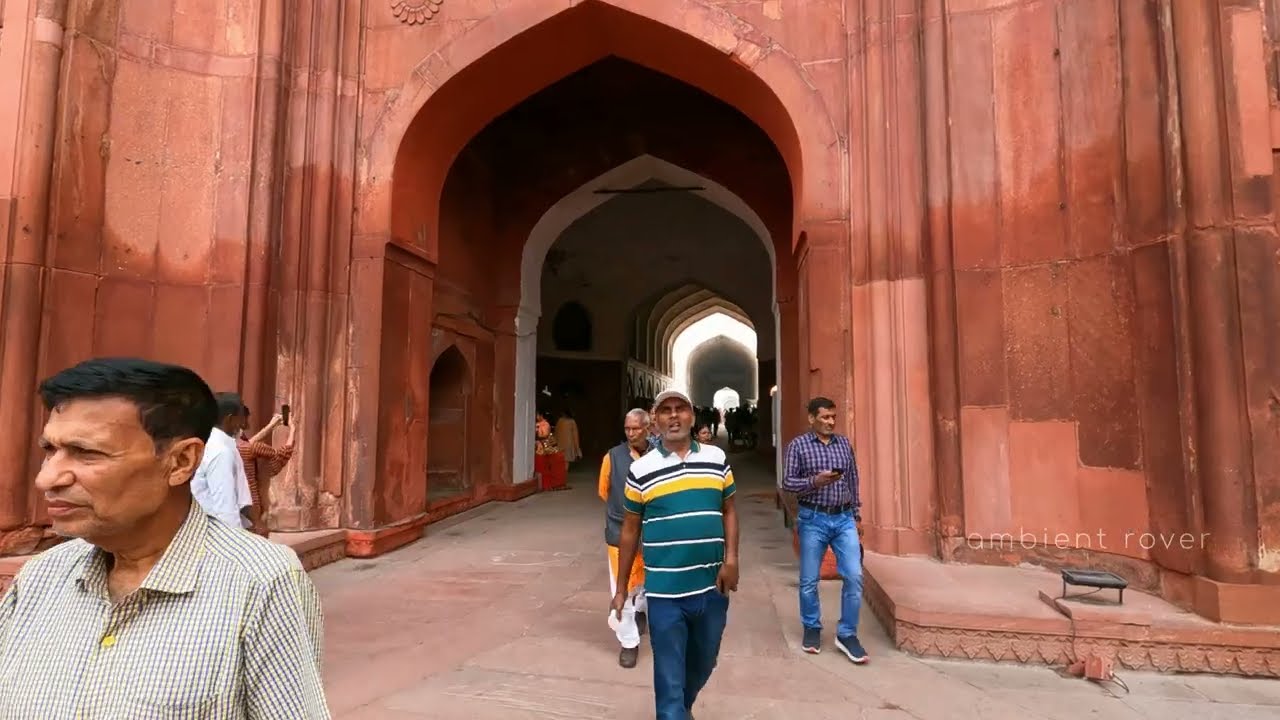A bustling horizontal rectangular image captures a group of people navigating in and out of an ancient, reddish stone or concrete structure resembling a temple or important monument, which likely serves as a tourist attraction. The structure features prominent and non-perfectly rounded archways, leading into a spacious, darker room with a similar arched opening on the other side, suggesting an exit. Vibrant colors adorn the crowd, with individuals in shades of blues, purples, greens, yellows, blacks, whites, and oranges. In the foreground, a man with short brown hair, darker skin, and a checked button-down shirt stands on the lower left, while another man in a striped blue, yellow, green, and white polo shirt with blue jeans faces the camera directly. Behind him is another man with short, graying hair in a yellow shirt and gray jacket. Another man to the right wears jeans, tennis shoes, and a plaid button-down shirt. Most people appear to be men, possibly Indian, and some are busy taking photographs. The image's bottom right corner displays the text "ambient rover."